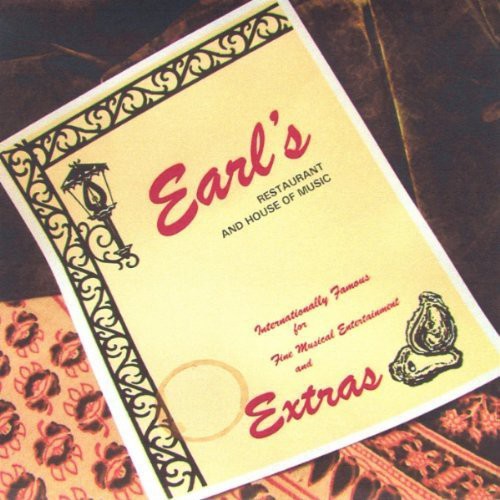The image depicts a weathered restaurant menu, possibly from the 70s or 80s, labeled "Earl's Restaurant and House of Music." The name "Earl's" is prominently displayed at the top in bold red cursive letters, while "Restaurant and House of Music" is printed below in black text. At the bottom, additional red cursive text announces, "Internationally famous for our musical entertainment and extras." Next to this text, there is an illustration of oysters. Surrounding the menu, a decorative black scroll-like border features an old-fashioned outdoor lamp at the sides and top. The white menu itself shows signs of age, including a visible brown coffee mug stain on the lower left corner. The background consists of a dark brown wooden surface, partially covered by a psychedelic floral-patterned fabric, adding a vibrant and nostalgic touch to the scene with hues of red and yellow. The menu appears slightly askew in the image.